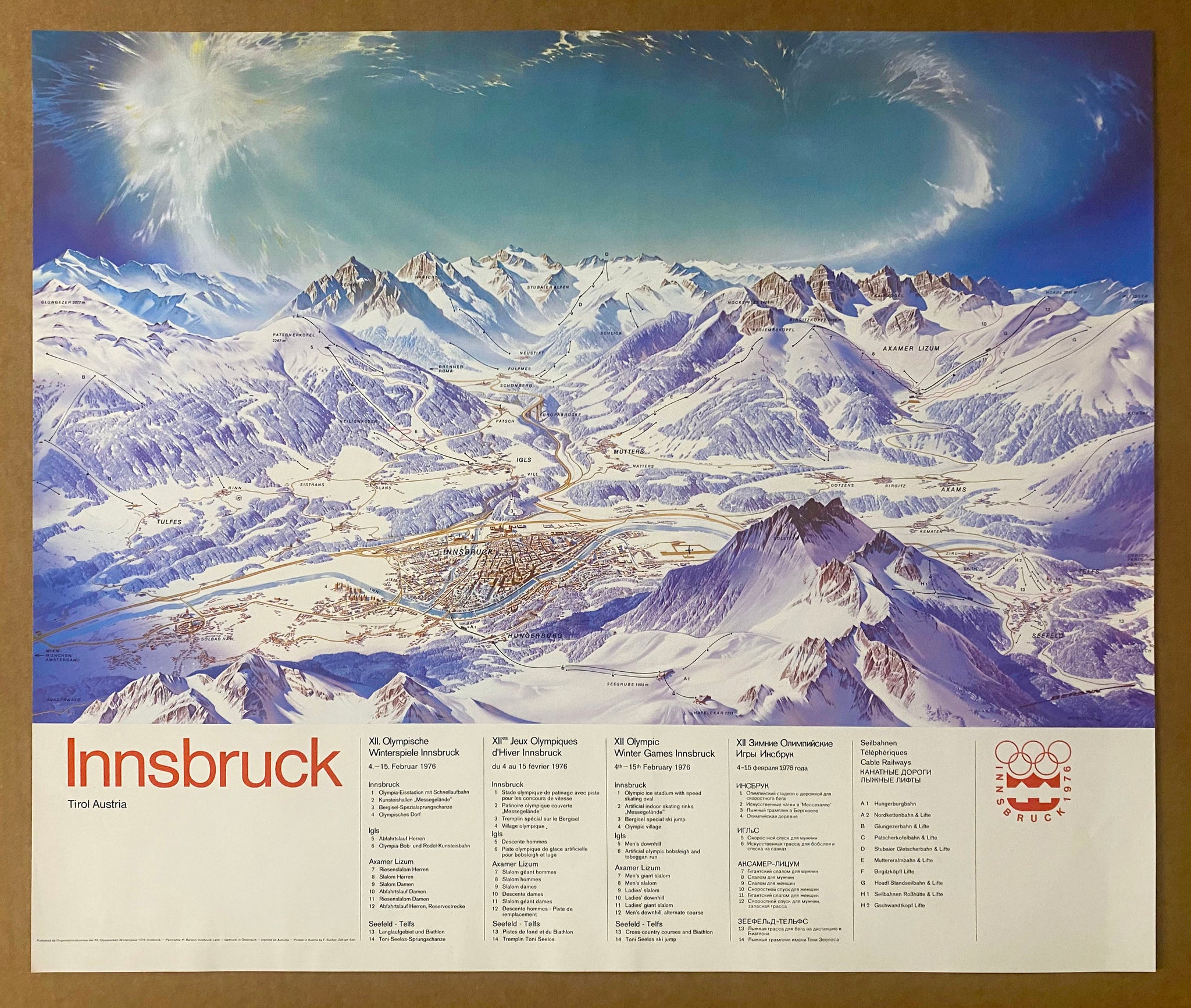This is a framed poster prominently featuring a vivid illustration of a snow-covered mountainous region, likely the Alps, with a picturesque ski town nestled in the foothills. The upper two-thirds of the image showcase the majestic mountains and an expansive, mesmerizing sky illuminated with teal hues and splotches of white light, reminiscent of an aurora borealis. Dark blue shades add depth to the sky, complementing the serene landscape. Ski tracks and routes are evident, descending from the mountain peaks to the village below. The poster is bordered by a thin brown frame that encloses the artwork elegantly.

The bottom quarter of the poster, on a tan background, clearly displays the word "Innsbruck" in bold red letters, indicating the location, while just underneath, smaller text likely reads "Tirol, Austria." To the right of this text, the Olympic symbol is prominently shown alongside dark red magenta logos and the text "Innsbruck 1976," signifying the 1976 Winter Olympics. Additionally, the bottom section contains five columns of smaller text with bold headings, seemingly detailing the events or various ski tracks related to the Olympics.

Overall, this detailed and vibrant poster beautifully captures the essence of Innsbruck and its role in the 1976 Winter Olympics, combining artistic illustration with informative text.